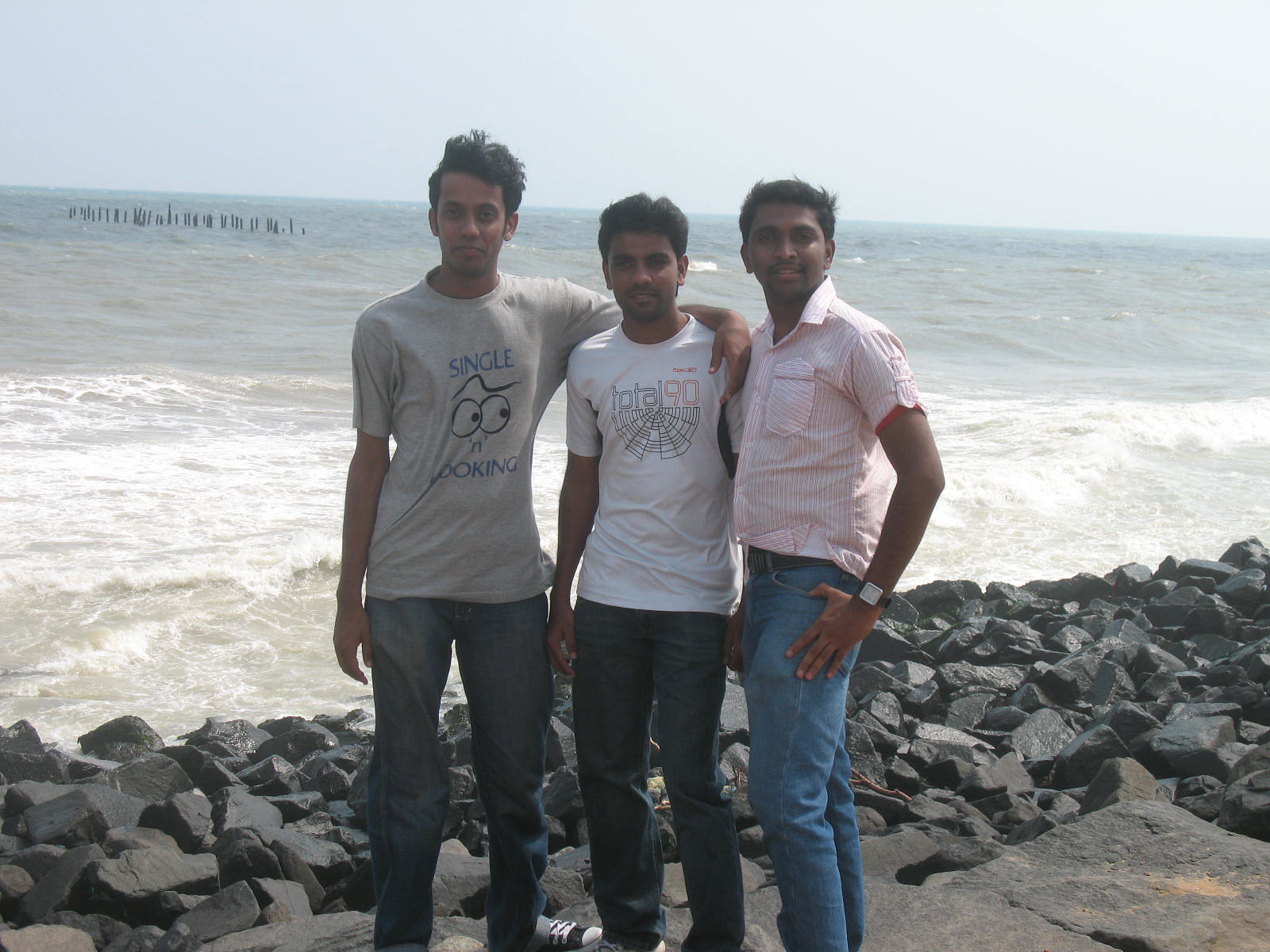This horizontally aligned rectangular image features three young Indian men standing on a rocky shoreline by the ocean. The foreground shows them posed on large black rocks, which gradually transition into smaller rocks closer to the water. The waves in the background exhibit white tips, with the shallow water appearing murky green, and the horizon blending into a bluish-gray.

The man on the left is dressed in dark jeans and a grey t-shirt that has the phrase "Single and Looking" with eyeball graphics in the center. His short, thick hair is windblown, adding a touch of casualness to his appearance. He has his arm around the man in the middle, who is shorter and sports a white t-shirt with the caption "PLA 90" (or "total 90") and a spider web print beneath it. He is also wearing dark blue jeans and has short, brown hair with light facial hair.

To the right, the third man stands out with a slightly more formal look. He wears a tucked-in red and white striped button-down shirt with a pocket, complemented by lighter blue jeans and a leather belt. His short brown hair and thin facial hair, along with a watch on his left wrist, complete his ensemble. All three appear to be in their twenties, enjoying a moment together by the sea.